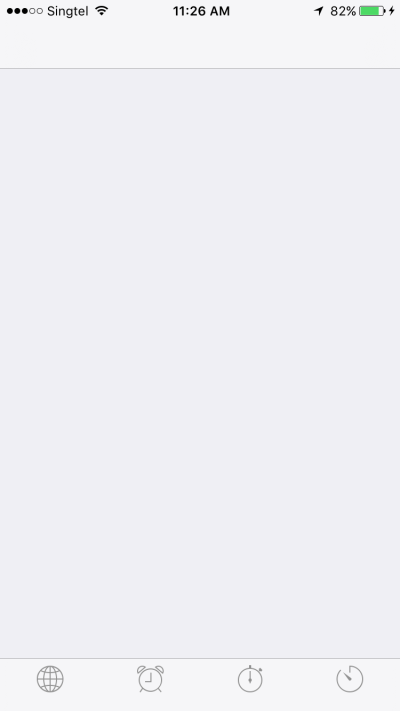A detailed screenshot of a smartphone display, featuring a sleek gray background. At the top of the screen, the telecommunications provider "SingTel" is listed, with a full signal bar. The current time is displayed as 11:26 AM, and the battery is at 82%. Below the top status bar, there are three filled black dots and two empty dots, all aligned horizontally.

The central part of the screen is predominantly gray, transitioning to a lighter gray shade towards the bottom. In the lower portion, several small icons are visible. The first icon is a globe, followed by an alarm clock symbol. The next icon resembles a traditional clock face, with dots indicating the 12 and 1 positions and a single hand. The final icon is also a circular clock face, but this one is missing a segment between the 11 and 12 marks. The clock hand in this icon points toward the 11.

The overall image is minimalistic, emphasizing the status indicators and icons against a subtle, gradient gray background.